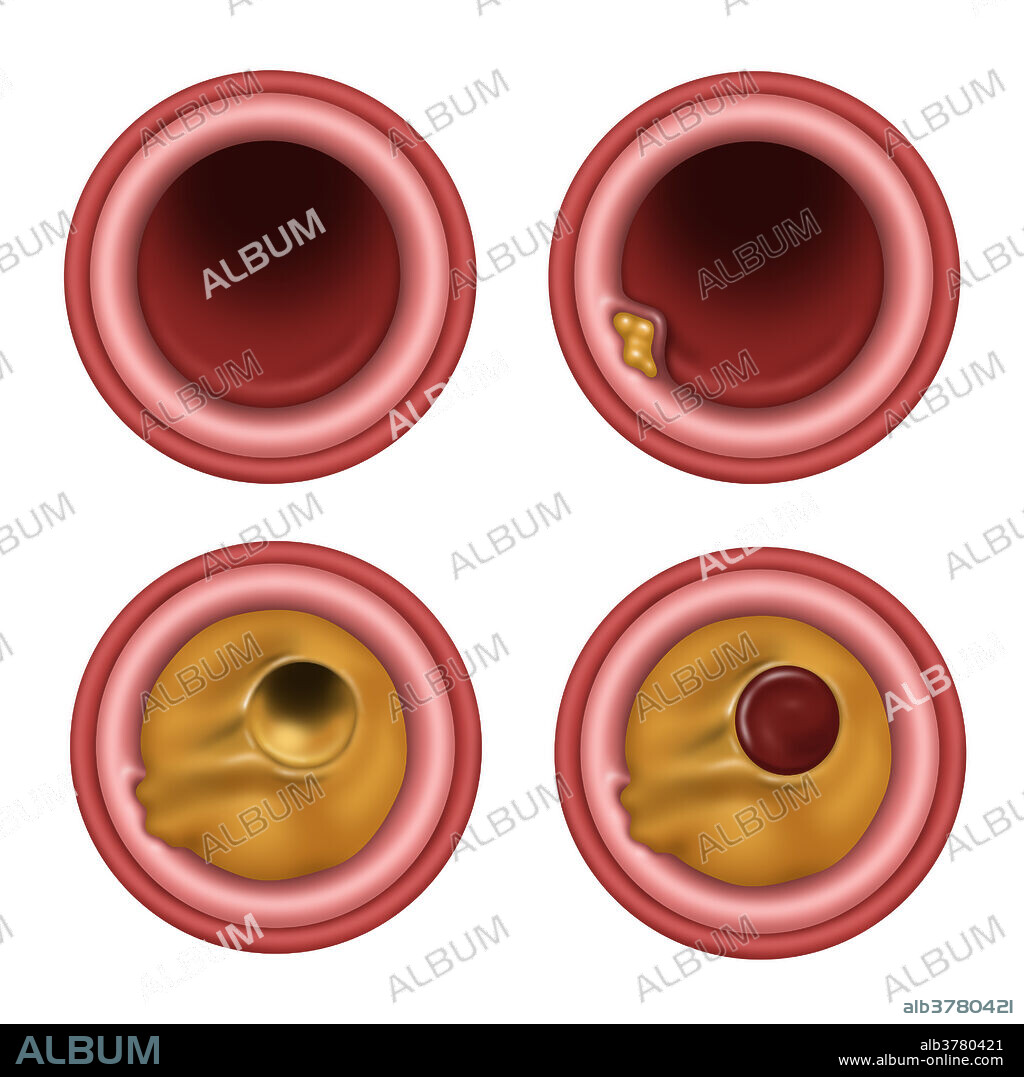This stock photo, watermarked diagonally with "ALBUM album," features a series of four abstract circles arranged in a 2x2 grid. The upper two circles are visually akin, each featuring a dark peach brown outer rim, a lighter fleshy inner ring, and a hollow center with a dark reddish-brown tone. The circle on the upper left, however, has a distinct bulge at the eight o'clock position filled with a bubbly gold fluid, suggesting an abscess.

Below these, the lower two circles maintain the same rim structures but differ internally. The left circle's center is filled with a gold liquid, which itself contains a smaller hollow circle. The right circle mirrors this, except the small circle within the gold liquid is now filled with a reddish-brown fluid, contrasting with its counterpart.

A thin black banner at the bottom of the image carries the text "album" in blue on the left and small white text "ALB 3 7 8 0 4 2 1 www.album-online.com" on the right, repeated in gray text above. The repeated watermark "album" and the specific branding details suggest a connection to the website www.album-online.com, although the image remains abstract, with enigmatic circular designs and unclear thematics.